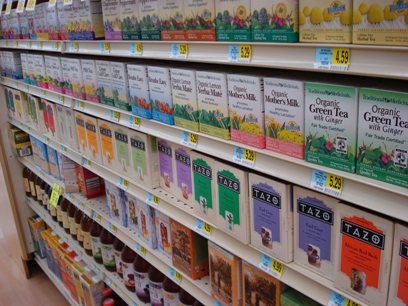This is a color photograph of the tea aisle in a grocery store, showcasing six shelves fully stocked with a variety of teas, including numerous organic options and several brands such as Tazo. The shelves display an array of brightly colored boxes, each representing different flavors. Prominent boxes include labels like "Organic Mother's Milk" and "Organic Green Tea with Ginger." On the top shelf, there is a tea box adorned with pictures of fruit, with price tags visible across the shelves, listing prices such as $4.59, $5.29, and $4.99. At the very bottom of the display, there are some jar containers and bottles of juice, distinct from the tea selection above. The yellow price tags, in addition to blue tags beside them, draw attention to the various costs of the teas on offer.